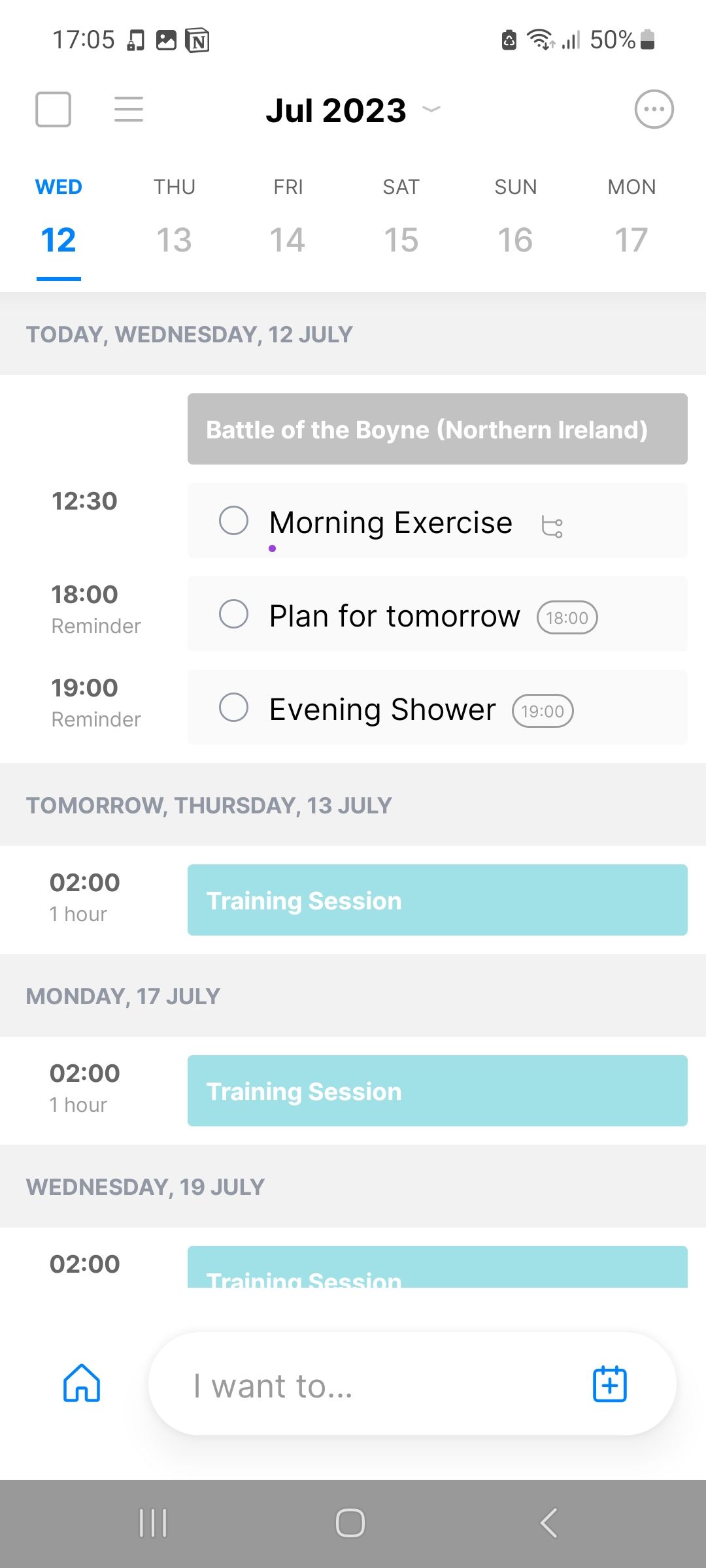Screenshot Description:

The image appears to be a screenshot taken from an Android device. The screen has a white background with black text at the top, displaying the time as 17:05. Below the time, there is an icon of a device resembling another phone with a lock on it and the Instagram logo next to it. A 3D square with an 'N' in it is shown, the purpose of which is unclear. 

The screenshot indicates the device is in power saver mode, with a fully charged battery and full Wi-Fi signal strength (3 out of 4 bars). The phone battery is at 50%, which is also displayed prominently. 

There is a grey square marked with the abbreviation "JUL," signifying July 23. On the right, there's a circular button with three vertical dots.

The image continues with a blue highlighted date, "Wed, 12," indicating Wednesday, 12 July. Below this, the days are listed in black text at the top and grey text at the bottom from "Thurs, 13" to "Mon, 17."

A section highlighted in grey indicates "Today, Wednesday, 12 July," followed by a schedule:

- 12:30 - Morning exercises
- 18:00 - Plan for tomorrow
- 19:00 - Evening showers (with a reminder to shower)

Additional notes for the week's schedule include training sessions mentioned for "Thursday, Monday, and Wednesday" marked with "O2."

At the bottom of the screenshot, there is a grey bar with three vertical lines on the left, a square in the center, and a back arrow pointing to the left on the right side.